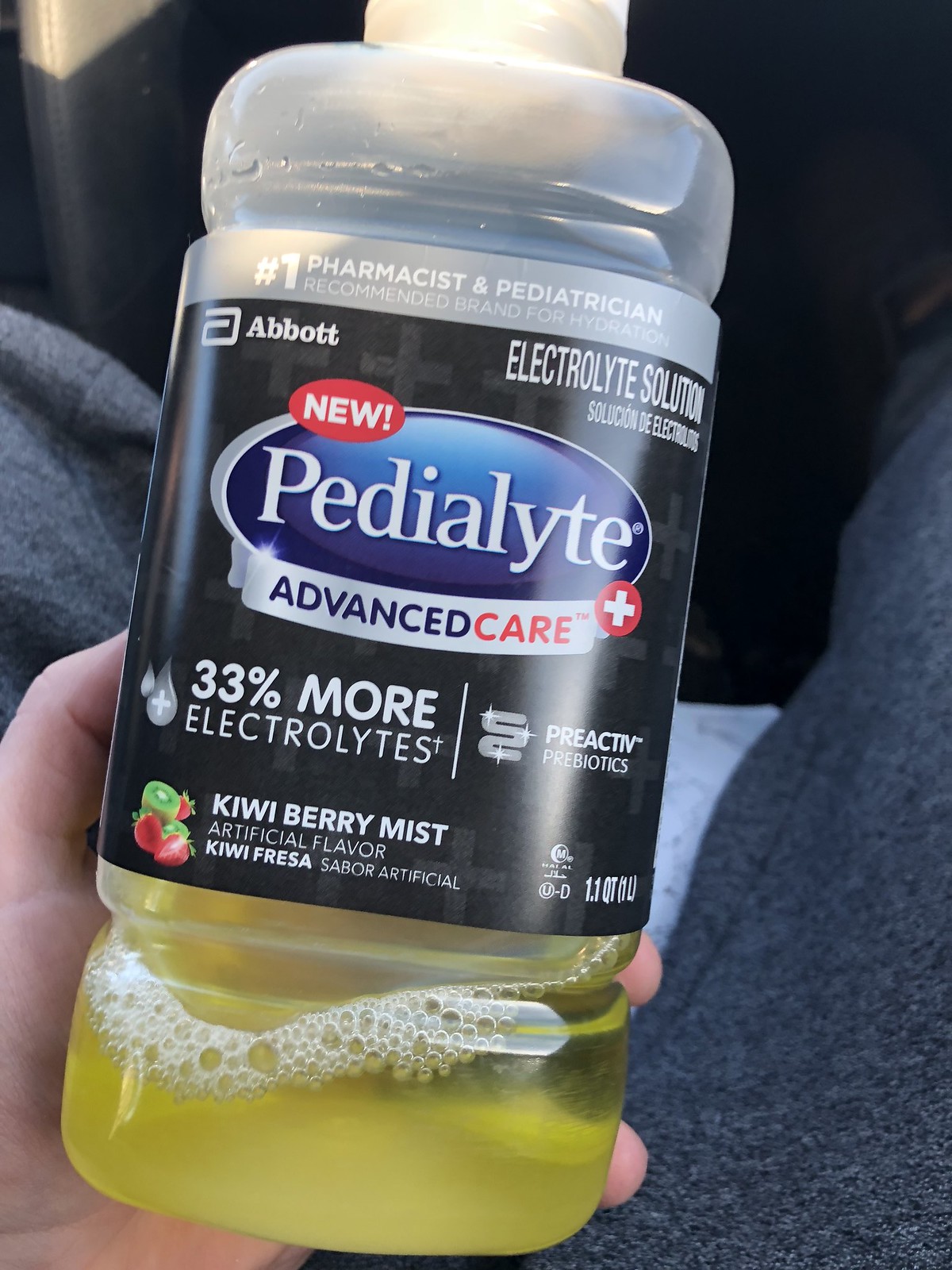The photograph captures a close-up, vertical, first-person perspective of someone holding a nearly empty clear plastic bottle in their left hand, featuring a yellow liquid with frothy white bubbles. In the background, you can see the person's legs clad in slightly baggy grey pants, suggesting they are sitting down. The label around the middle of the bottle is primarily black with a detailed layout: at the top, a silver base with the phrase "#1 Pharmacist and Pediatrician Recommended Brand for Hydration" is prominently displayed. The upper left corner of the black label bears the Abbott logo, while the upper right corner states "Electrolyte Solution," also translated into French. The center features a blue oval with the white text "Pedialyte," accompanied by a red oval marked "New," and further below, "Advanced Care Plus" with a trademark symbol. The label also highlights that the product contains "33% more electrolytes." At the bottom, the flavor "Kiwi Berry Mist Artificial Flavor" is mentioned alongside a small graphic of kiwi and berries.